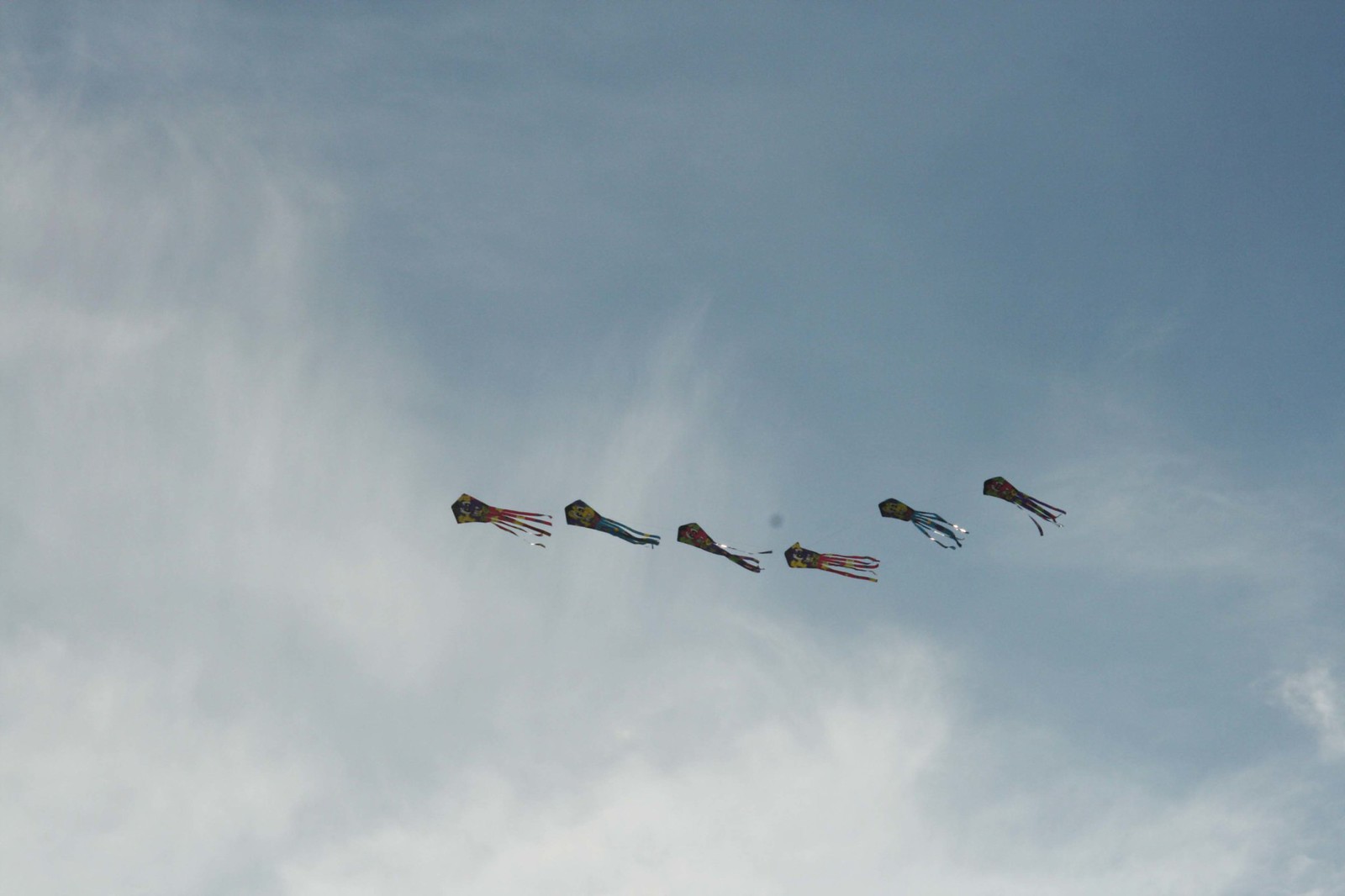Against a backdrop of a pale blue sky dotted with wispy, cotton-like cirrus clouds, six kites soar gracefully in a slightly diagonal line across the middle of the frame. The sky is clearer in the upper right-hand corner, with thicker clouds towards the bottom left, creating a picturesque setting. The kites, maintaining traditional kite shapes, appear grouped closer together, possibly tied to the same string, given their tight formation. They exhibit a vibrant array of colors: reds, blues, yellows, purples, and blacks, with some even reflecting a shiny, plastic-like material as sunlight glints off their surfaces. Each kite features fringed tails that flutter elegantly in the breeze. The first and fourth kites proudly display red tassels, while blue and darker tassels adorn the others, adding to the spectacle. Despite the strings being invisible, one can deduce a coordinated effort behind this aerial display. The kites' orientation—with the thicker part pointed to the left—adds dynamic movement to the serene sky scene.